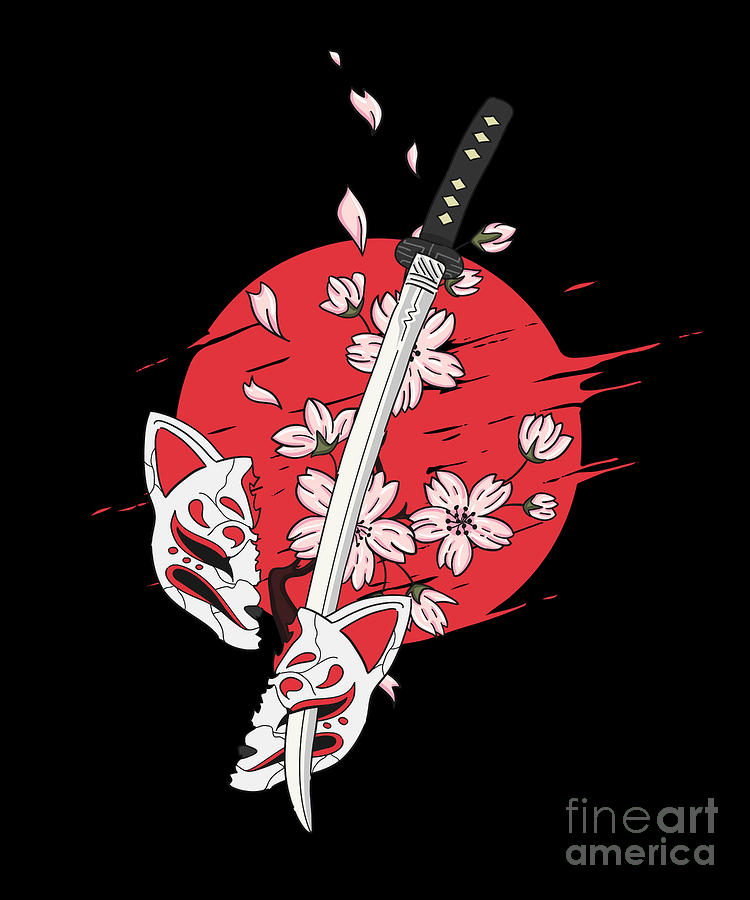This Japanese-style artwork features an intricate design on a black background, prominently displaying a red circle reminiscent of Japan's flag. At the bottom of the image, "Fine Art America" is inscribed in gray. Central to the composition is a white and gray katana sword with a black handle adorned with six gold diamonds. The katana dramatically slashes through a traditional Japanese cat mask, splitting it in half. The mask is white with red accents on the ears, slanted eyes, and mouth. Surrounding the scene, pink Sakura flowers and petals elegantly drift across the circle, adding a touch of grace. The red circle itself bears several slashes, symbolizing dynamic movement, and is accompanied by branches from which the blossoms seem to originate. This animated-style poster effectively captures the essence of Japanese art and culture.